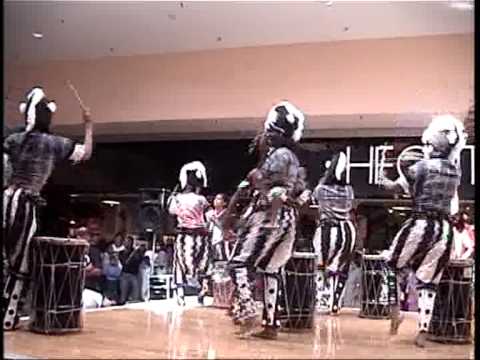The photograph captures an energetic performance of an African musical and dance ensemble in an indoor auditorium with a raised, highly polished stage reflecting light from a visible spotlight on the white ceiling. The performers, identified as Atilogu dancers, number around six and are dressed in elaborate costumes. These include grey shirts and white belts over black and white striped trousers that are baggy at the top and tight at the bottom, paired with polka-dot elements and an additional skirt-like garment over the trousers. Each dancer dons a distinctive helmet adorned with white feathers forming a mohawk-like structure, complemented by two white dots on either side resembling small ears. Large, strategically placed drums, standing just above knee level, accompany the dancers on stage. Despite the picture's slight blurriness, the enthusiastic audience's laughter and cheering are evident, suggesting a lively and engaging performance. The scene is well-lit, likely due to the strategically placed spotlights and speaker stands hinting at audio support in the background. One particular dancer is seen holding an object above his head, potentially a drumstick, possibly indicating his role in orchestrating the group's rhythm and movements.